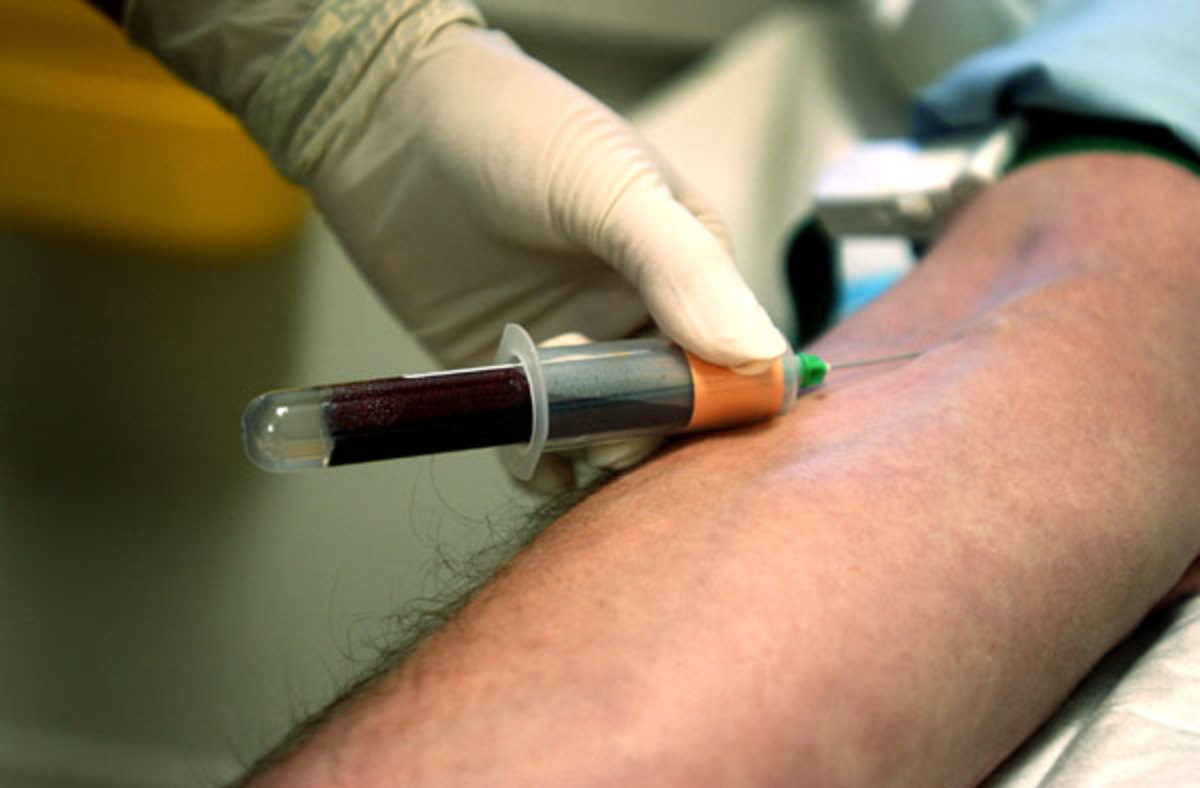The image captures a detailed scene of a medical procedure where blood is drawn from a patient's left arm. The arm, outstretched and resting on a surface, is relatively hairy with dark, skinny hairs, indicating the patient has a lighter skin tone. The focus is on a needle inserted into the vein located in the crease of the arm. A medical professional’s gloved hand, wearing a white rubber glove, holds the syringe. The needle has a green tip, and the syringe features an orange band around its middle, containing a glass vial filled with dark red blood, suggesting a significant volume, possibly more than 20 ml. The professional's thumb is on the top of the syringe while the other fingers are positioned against the patient's skin. The background is blurry, suggesting an office setting, with indistinct objects visible, including a yellow trash can and a sink.